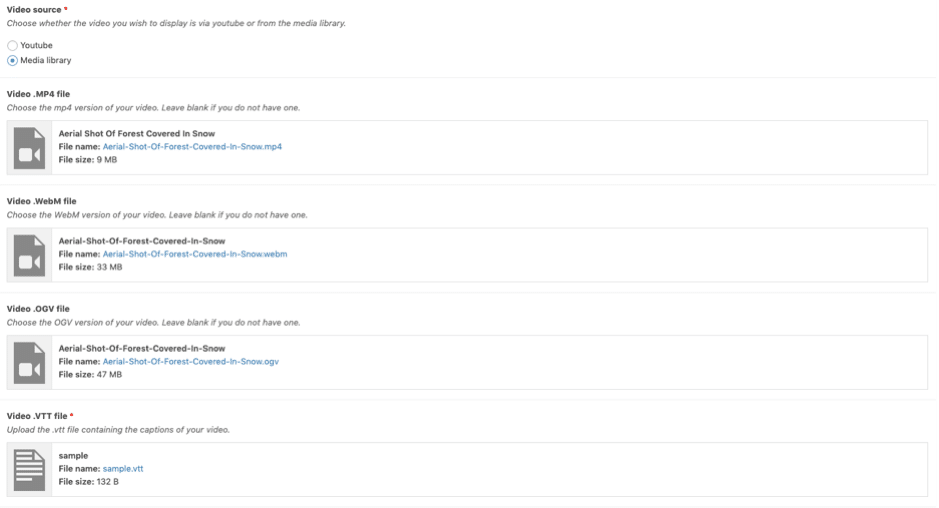The image shows a website settings page featuring a list of video files available for embedding. Each file is a version of the same video, titled "Aerial Shot of Forest Covered in Snow," presented in different formats: .mp4, .webm, and .ogv. The .mp4 file is the smallest, with a size of 9 megabytes, while the .webm and .ogv files are larger, at 33 and 47 megabytes, respectively. A header labeled "Video Source" instructs users to choose whether the video should be displayed via YouTube or from the media library. In this instance, "Media Library" is selected, resulting in the display of these video file options for embedding into a website.